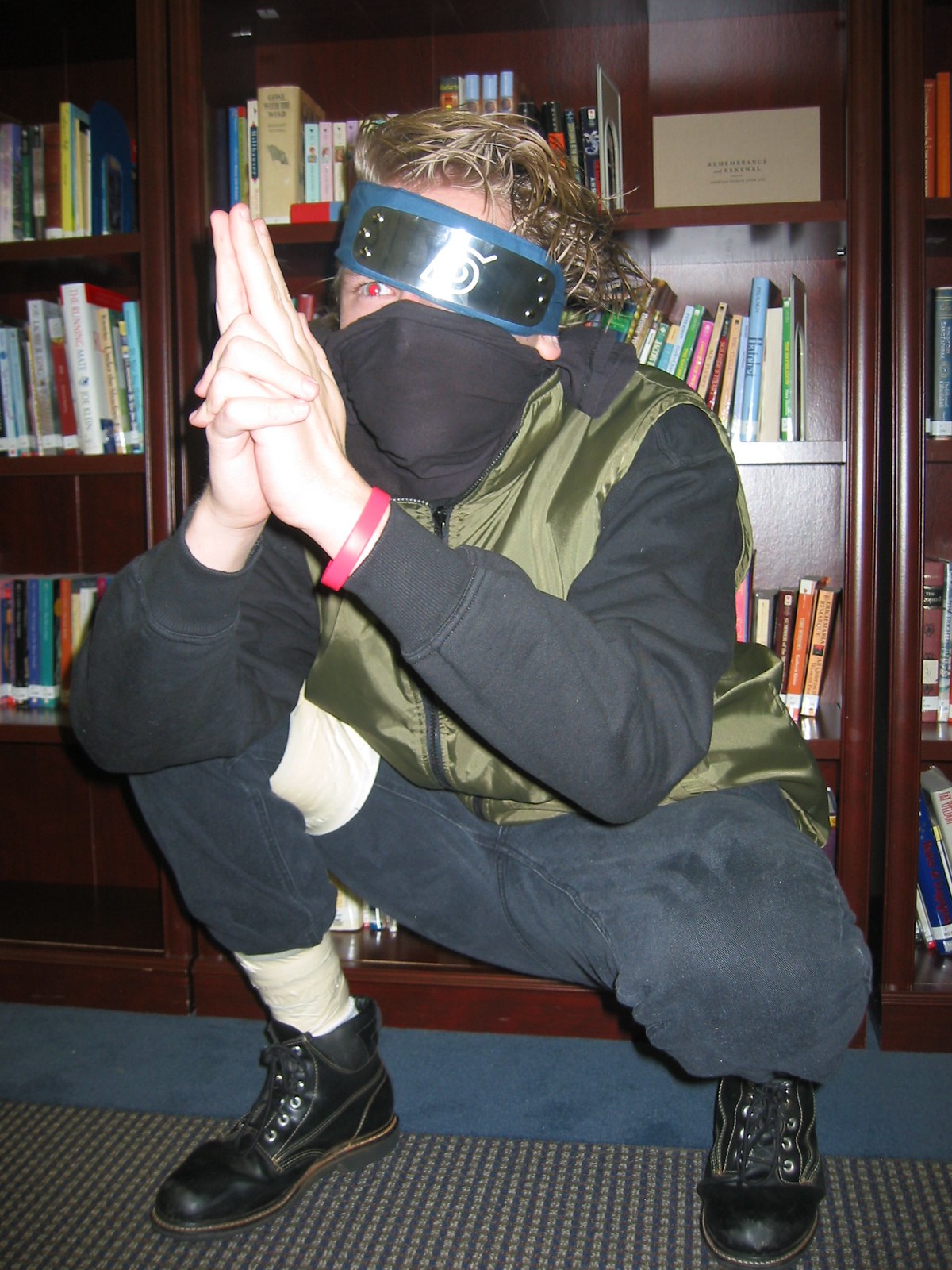In a portrait-oriented photograph taken indoors, a young Caucasian man is depicted cosplaying as a character from the manga Naruto. The backdrop consists of dark wooden bookshelves filled with books, suggesting a library setting. The floor features a blue and tan patterned carpet. The man, who has semi-long blond hair reaching his ears, is squatting in front of the bookshelves. He is dressed in a distinctive outfit: a green vest over a black long-sleeved shirt, dark blue jeans or pants, and black boots. White socks or bandages are wrapped around his ankles. He is also wearing a black face mask and has a blue bandana tied around his head, pulled down over one eye, revealing his red-tinted left eye. He has a red wristband on one wrist, and his hands are clasped together in front of him, with the first two fingers pointing up, mimicking a special ninja sign from the series. Goggles are positioned sideways on his head. The detailed pose and attire indicate he’s emulating a specific Naruto character with considerable effort.